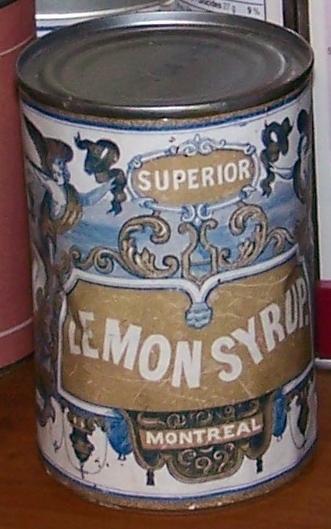The image showcases a close-up view of a vintage can with a dated, antique quality. The can's design evokes French styling reminiscent of something from Versailles, characterized by its sophisticated and aged label. The label is primarily white with a bluish tinge and features some indistinct artwork that adds to the classical feel. Centrally positioned at the top of the can, within a brownish-tan oval, the word "Superior" is printed in white lettering. Directly beneath, against a larger brown rectangular background, "Lemon Syrup" is also displayed in white letters. Further down, a smaller narrow brown rectangle highlights "Montreal," reinforcing its association with a French heritage. The photo itself is a bit blurry and unfocused, lacking sharpness, but the details on the label are mostly readable. The entire presentation suggests an antique item, possibly discovered in an old cabinet or home, emphasizing its historical and aesthetic value.